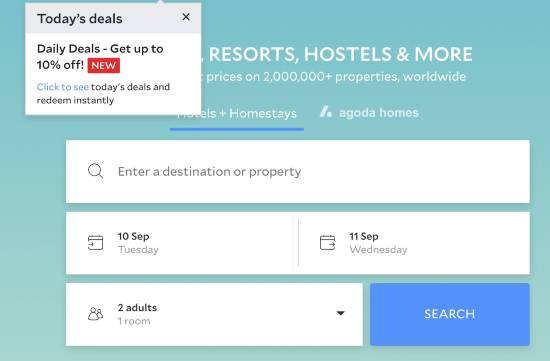The image depicts the homepage of a website likely named "Odell's," featuring various travel and accommodation options. Prominently, a square pop-up labeled "Today's Deals" overlays the page, advertising daily discounts of up to 10%. This pop-up includes a striking red box with white text reading "New," and a blue hyperlink stating "Click to See." Below this, in black text, it announces "Today's Deals and Redeemed Instantly," with a clickable 'X' to close the pop-up and reveal more of the page.

The main webpage, partially obscured by the pop-up, features a top header that reads, "Resort, Hostels, and More, Prices on 2 Million Pressed Properties Worldwide," though part of this text is cut off. Under this header, a selection bar indicates "Hotels and Homestays" with a blue underline confirming this choice. There is also an icon resembling two thick lines forming a triangle with the option text "Go to Homes."

Beneath the selection bar, a prominent search box invites users to "Enter Destination or Property." Below this, two smaller boxes likely meant for inputting check-in and check-out dates display pre-selected dates: September 10th (Tuesday) and September 11th (Wednesday). Additionally, a dropdown menu allows users to modify their selections for the number of rooms and guests, which currently shows "two rooms, one adult." Finally, a search button at the bottom allows users to initiate the search based on their chosen criteria.